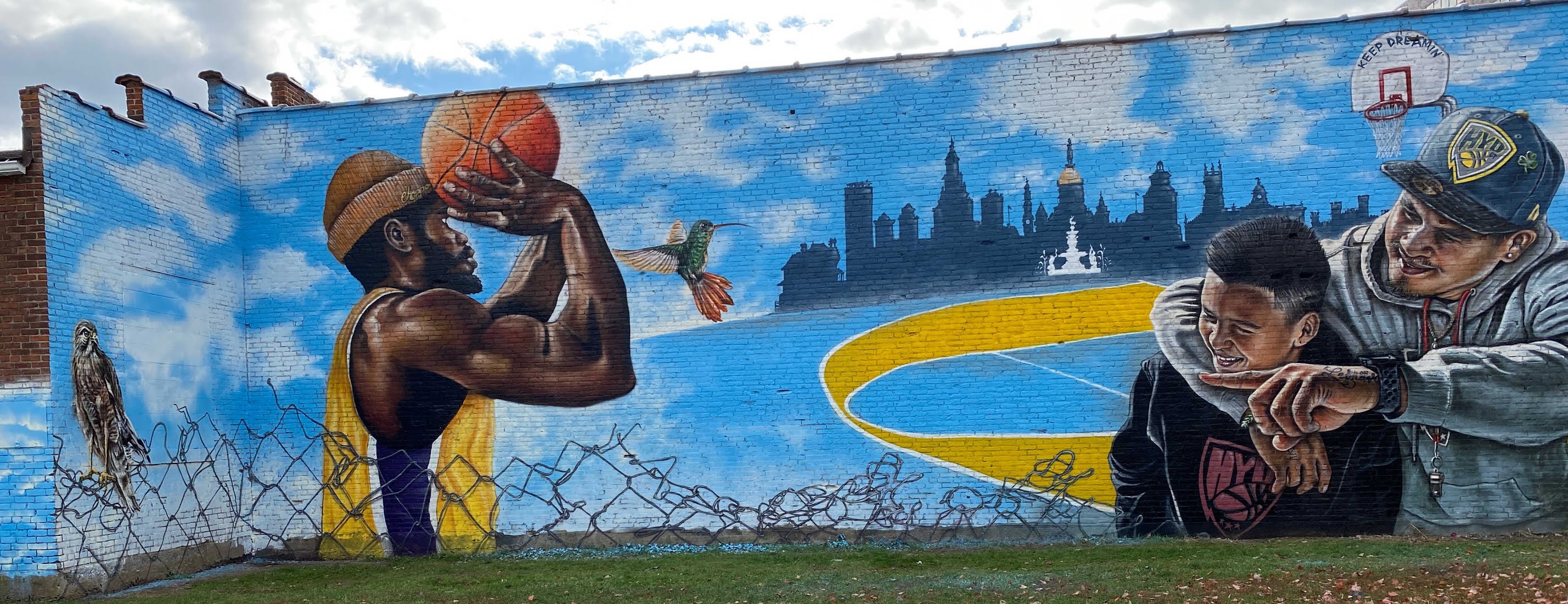This vibrant mural, painted on a large building wall, captures a dynamic scene set against a deep blue sky filled with puffy white clouds and silhouetted city buildings in the background. On the left-hand side, a black basketball player is depicted mid-motion, as if preparing to make a free throw. He wears a yellow and purple jersey, seen from a side view, and holds a basketball in both hands. A hummingbird flutters in front of him, while a hawk soars behind him.

Dominating the right-hand side of the mural, a man in a gray sweatshirt and hat is engaged in a joyful moment with a boy in a black sweatshirt who has a basketball design on it. The man has his arm around the boy's shoulder and is pointing towards the basketball player on the mural. Both are smiling and appear to be enjoying the scene. The mural incorporates a basketball court with a blue surface and a yellow arc. Near the basketball hoop, which is slightly off in the distance, there's a subtle lettering that reads "KEEP DUNKING." The topmost part of the mural features a gray patch of clouds blending into a clearer sky, enhancing the urban atmosphere of this lively and detailed artwork.